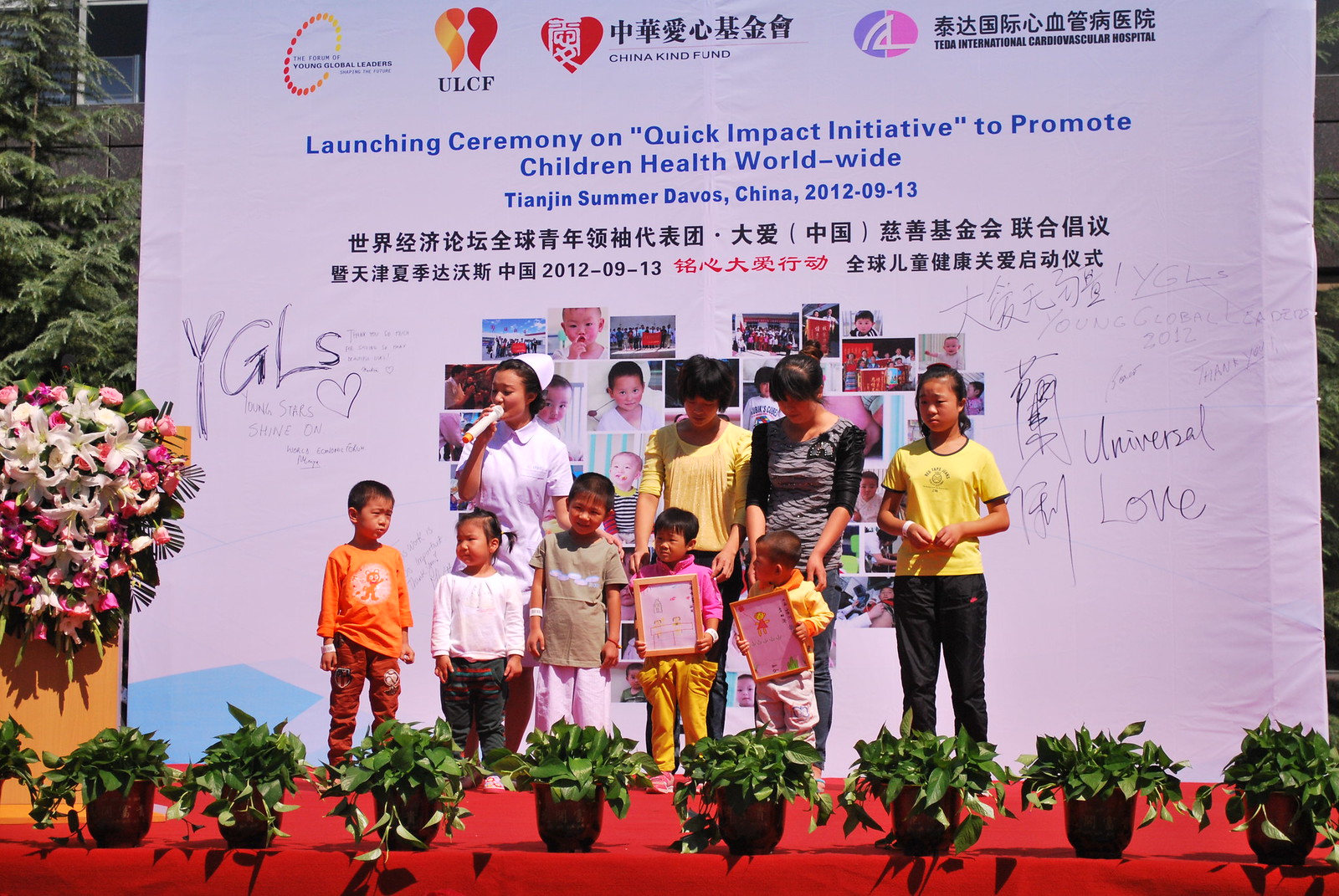This image captures the vibrant atmosphere of an outdoor celebration event, identified as the Launching Ceremony on Quick Impact Initiative to Promote Children's Health Worldwide. It took place in Tianjin, Summer Davos, China, on September 13, 2012. The red-carpeted stage hosts a diverse group of people, predominantly of Asian descent, comprising three adults, one teenager, and five children. Prominently featured are two children in the front row holding framed pictures. The stage is adorned with an array of potted plants with lush green leaves and a bouquet of pink and white flowers. Behind the group, a large white backdrop displays the event's title in blue font, along with various logos, including ULCF, China Kind Fund, and Universal Love. A nurse in a white uniform and hat stands to the left, speaking into a white microphone, surrounded by children who seem to be holding awards or pictures. The backdrop also features photos of potential participants or candidates involved in the initiative. The overall scene exudes a sense of unity and celebration, highlighting efforts to promote children's health globally.